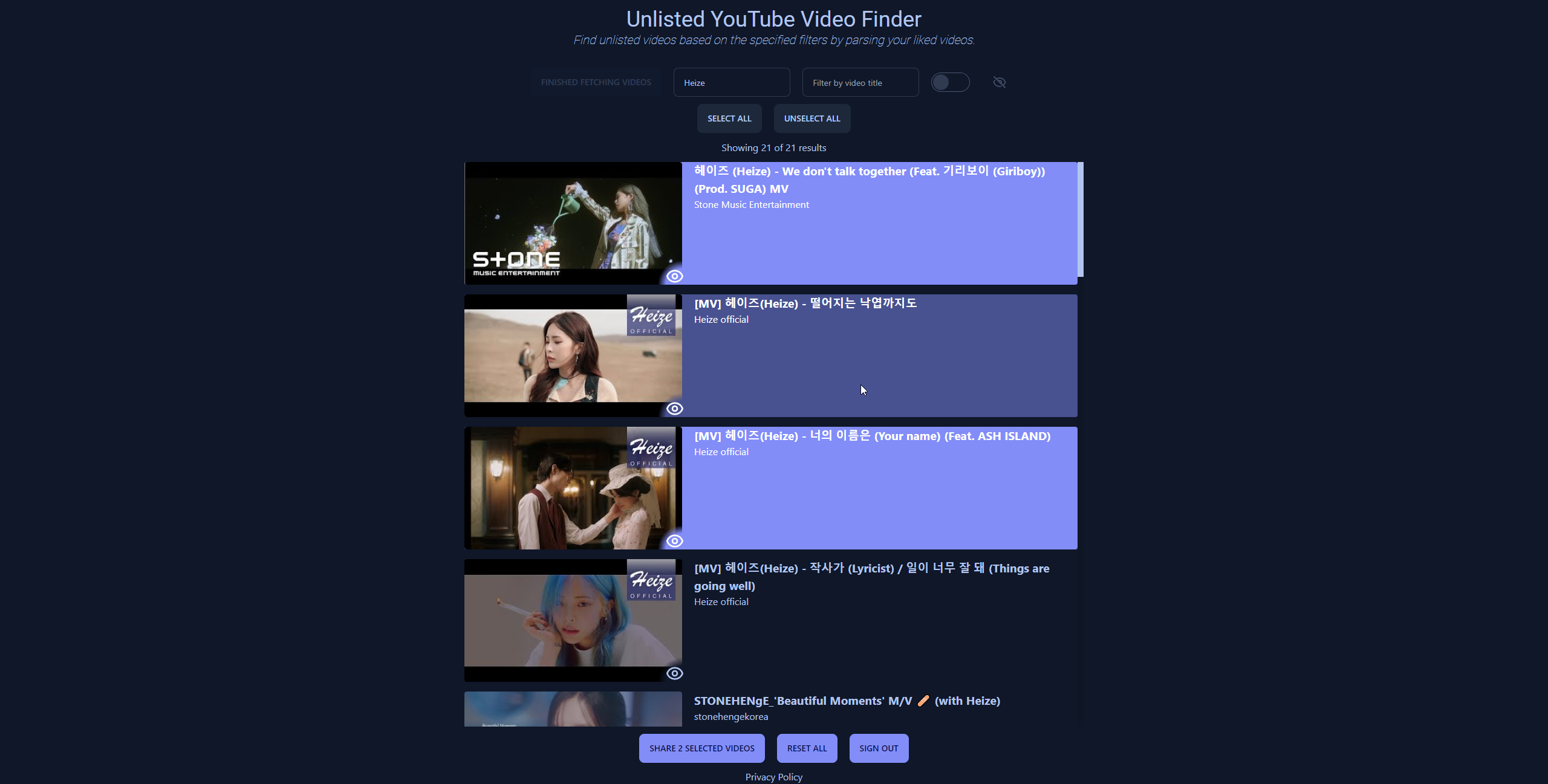This image displays a webpage titled "Unlisted YouTube Video Finder." The header explains the purpose of the tool: "Find unlisted videos based on the specified filters by parsing your liked videos." Below the header are several interactive elements, including search boxes and filter options.

Key features on the page include a button labeled "Finish Fetching Videos," and another box containing the word "Highs." There is a filter option titled "Filter by Video Title," and an on/off toggle switch that features an icon of an eye with a line through it, presumably to show or hide specific content. Additionally, there are buttons allowing the user to "Select All" or "Unselect All."

The interface displays a list of video results, showing "21 of 21 results." The videos are presented in distinctive purple-bordered boxes, each accompanied by a thumbnail image.

1. The first video, titled "Haze. We Don't Talk Together. Featuring Girl Boy. Proud Sugar MV," is from Stone Music Entertainment and features an image of a woman watering a flower.
2. The second video, simply labeled "MV, Haze," includes various characters in a foreign language and is from Haze Official. The thumbnail depicts a woman with brown hair in what appears to be a desert setting.
3. The third video is titled "Haze. Your Name. Featuring Ash Island. Haze Official" and shows a man and a woman in a scene from a music video.
4. The fourth video is named "Haze. Lyricist. Things Are Going Well," also from Haze Official, featuring an image of a woman with blue hair.

At the bottom of the webpage, there are buttons for further actions such as "Share to Selected Videos," "Reset All," or "Sign Out." The overall theme of the webpage is dark, predominantly using dark blue or black for the background.